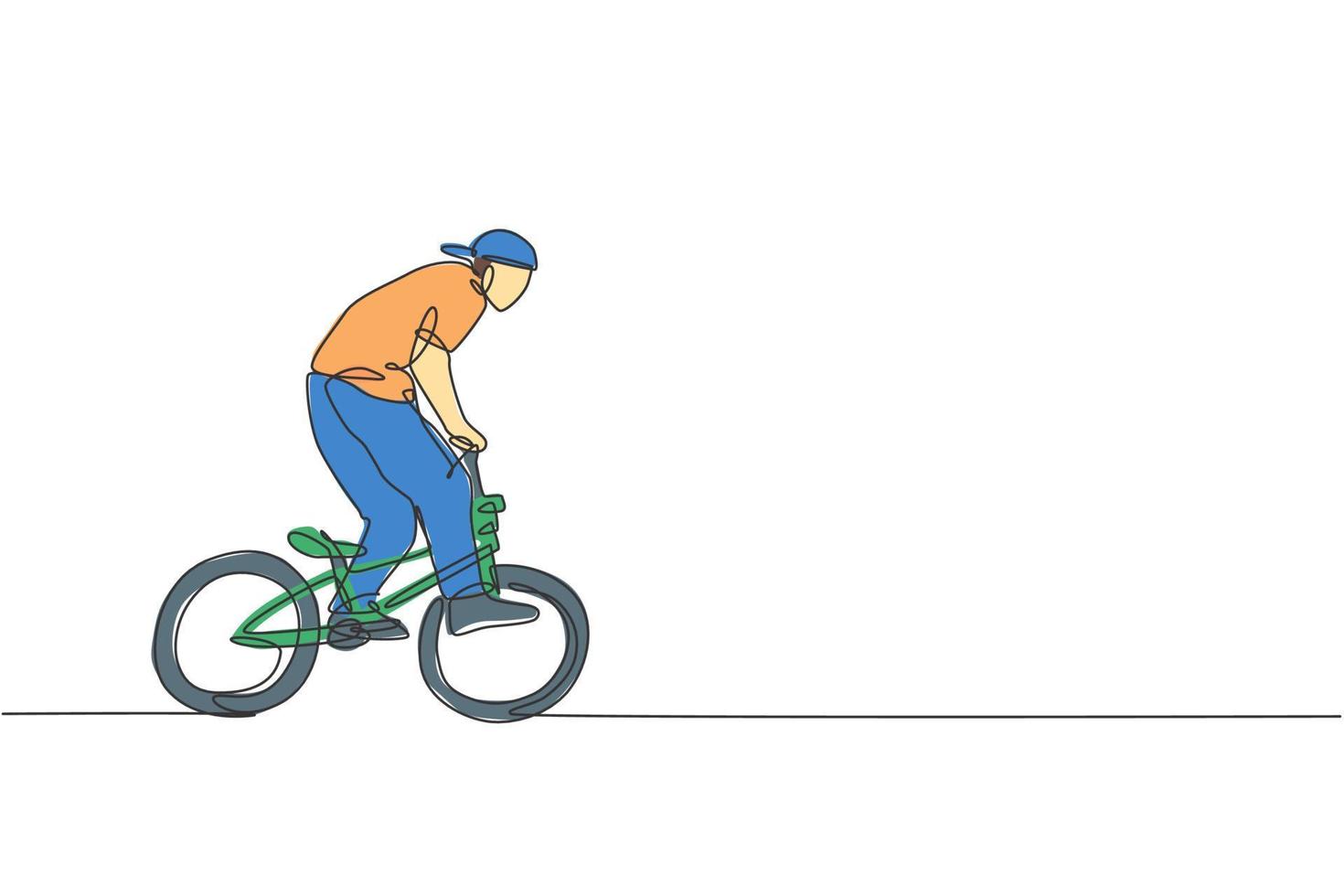The image is a two-dimensional, cartoon-style drawing set against a white background with a flat, black horizontal line representing the ground. The focal point of the drawing is a man riding a green bicycle that appears to be in motion, traveling from left to right. The man is depicted standing on one of the pedals while his other leg hovers in space, suggesting motion. He is not sitting on the bicycle seat but is instead positioned upright. His outfit consists of blue jeans, black shoes, an orange (or salmon-colored) shirt, and a blue backwards baseball cap. The man has white skin but lacks any detailed facial features or other distinguishing physical characteristics. The wheels and handlebars of the bicycle are dark gray or black. The image employs a continuous line drawing technique, giving it a unified and dynamic appearance.